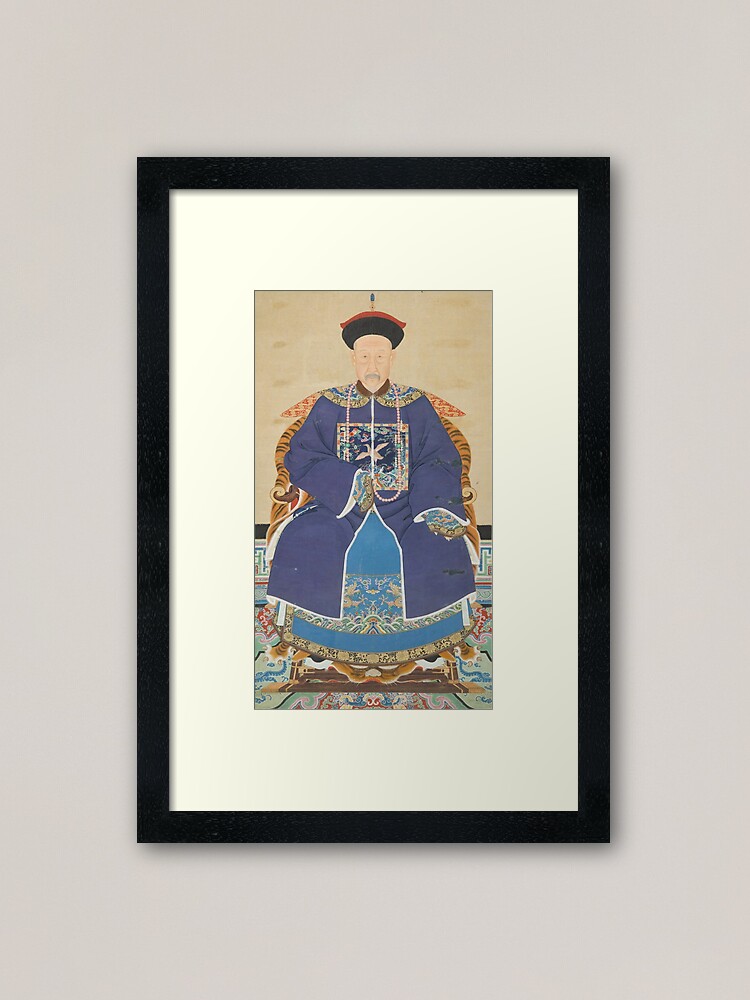This image is a framed picture displayed on a very light gray or off-white wall. The picture is within a sleek black frame and surrounded by a flat white mat. The artwork depicts an ornately dressed Chinese emperor sitting on a throne. The emperor is donned in a dark blue robe featuring an elaborate design of a flying crane or heron on the front and paired with a light blue skirt adorned with intricate patterns, though the exact details are hard to discern. He wears a striking black hat that widens towards the top, capped with touches of red, gold, and blue that come to a point. The throne he sits upon exhibits orange and black stripes reminiscent of tiger fur and is placed on an equally ornate carpet. The background of the painting showcases a tan wall, adding to the richness of the scene. This piece of art appears to be done with fine lines and delicate colors, possibly on rice paper, giving it a soft pastel appearance.